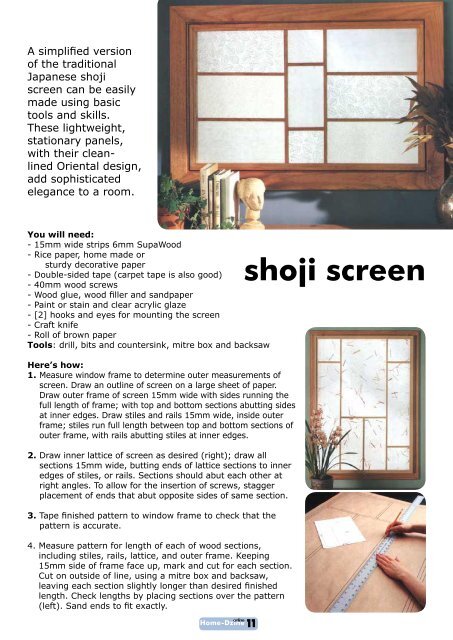This image serves as an instructional guide for creating a simplified version of a traditional Japanese shoji screen using basic tools and skills. The top section of the guide features a wood frame partitioned into three sections on the left, three smaller central sections, and three sections on the right, all containing square glass panels. Below, in bold black text, it’s labeled "Shoji Screen." The materials listed include 15mm wide wood strips, 6mm supawood, rice paper or sturdy decorative paper, various tapes, wood screws, glue, filler, sandpaper, paint or stain, clear acrylic glaze, two hooks and eyes, a craft knife, roller, brown paper, drill bits with countersink, a miter box, and a back saw. Step-by-step instructions detail measuring the window frame, drawing the screen outline on large paper, cutting and assembling the frame, stiles, rails, and lattice, ensuring precise fits by sanding, and finally checking the design accuracy against the window frame. Additional images at the bottom right illustrate the screen with possible debris or grass, the measuring process, and a decorative plant placed in front of the completed frame. These lightweight, stationary panels enhance a room with a touch of sophisticated, clean-lined elegance.